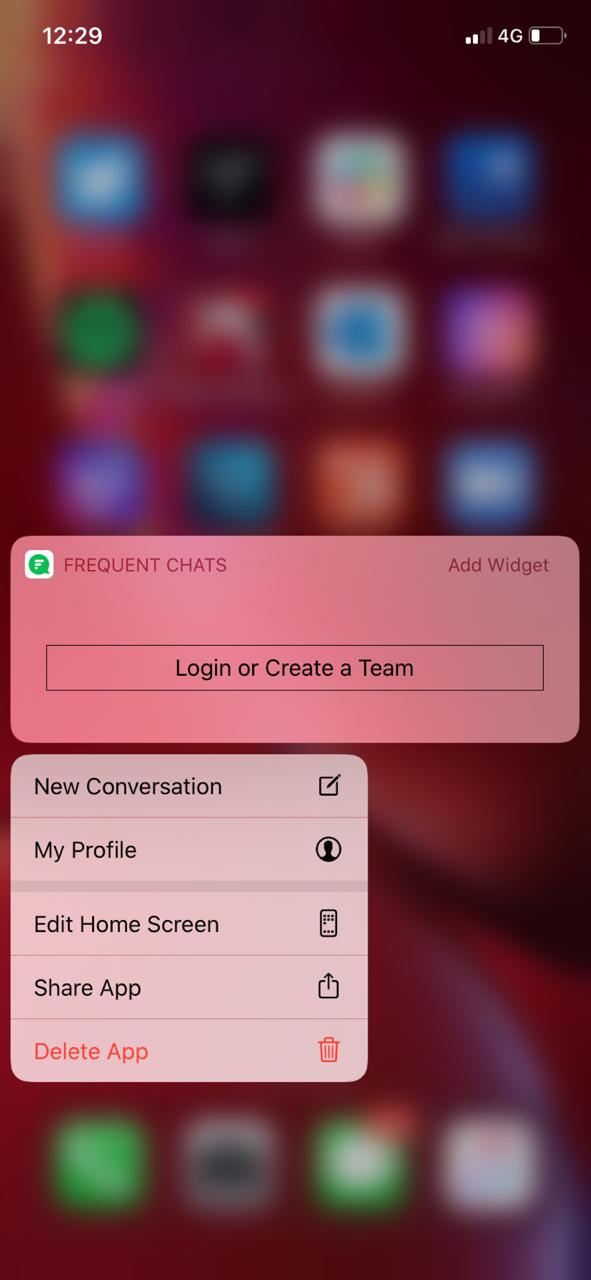The image is a screenshot taken from a cell phone. In the upper left corner, the time is displayed in white font as "12:29." Adjacent to it on the upper right, the cell phone reception icon shows only two bars alongside the "4G" indicator. Nearby, the battery icon is nearly depleted, hovering around 25%. The cell phone's background wallpaper is a reddish hue, partially obscured by a pop-up window, making the underlying icons appear blurred. 

The pop-up window prominently displays "Frequent Chats" in the upper left corner, accompanied by a white icon featuring a green speech bubble. On the upper right of this window, "Add Widget" is clearly visible. Within the pop-up, a conspicuous button reads "Log In or Create a Team," drawing attention as the central call-to-action in this interface.